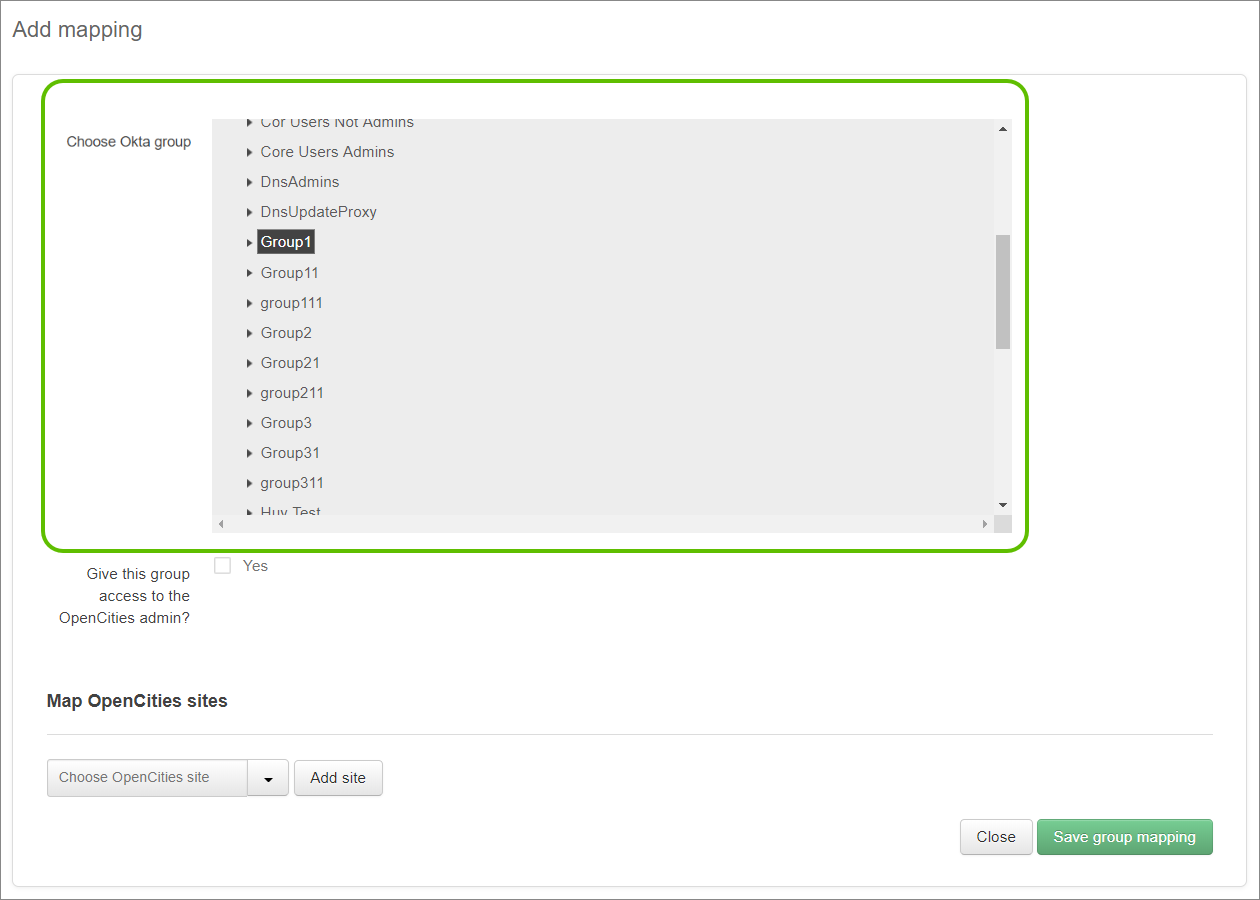This image is a detailed screenshot of a web page primarily composed of white background with black text and a notable green-encircled section towards the top. At the top of the page, the black text reads "Add Mapping". 

Below this header, an area encircled in green outlines the section titled "Choose Okta Group" (spelled O-K-T-A). Within this section, there is a gray rectangular area displaying a list of group names. These names include:

- Core Users not Admins
- Core Users Admins
- DNS Admins
- DNS Update Proxy
- Group 1 (highlighted in black)
- Group 11
- Group 111 
- Group 2
- Group 21
- Group 211
- Group 3
- Group 31
- Group 311

Below this list, part of the font is cut off, making the first word illegible, with the second word appearing to be "test". A scrollbar on the right suggests that additional items are listed but not visible in the current view. All the listings are bullet-pointed in black font against the gray background.

Beneath this section, the phrase "Give this group access to the OpenCities Admin" is displayed, accompanied by an unchecked checkbox labeled "Yes."

Further down, the text "Map OpenCities Sites" appears above a dropdown box labeled "Choose OpenCities Site" and a gray button that reads "Add Site".

In the lower right corner of the page, there is a "Close" button and a prominent, green button labeled "Save Group Mapping".